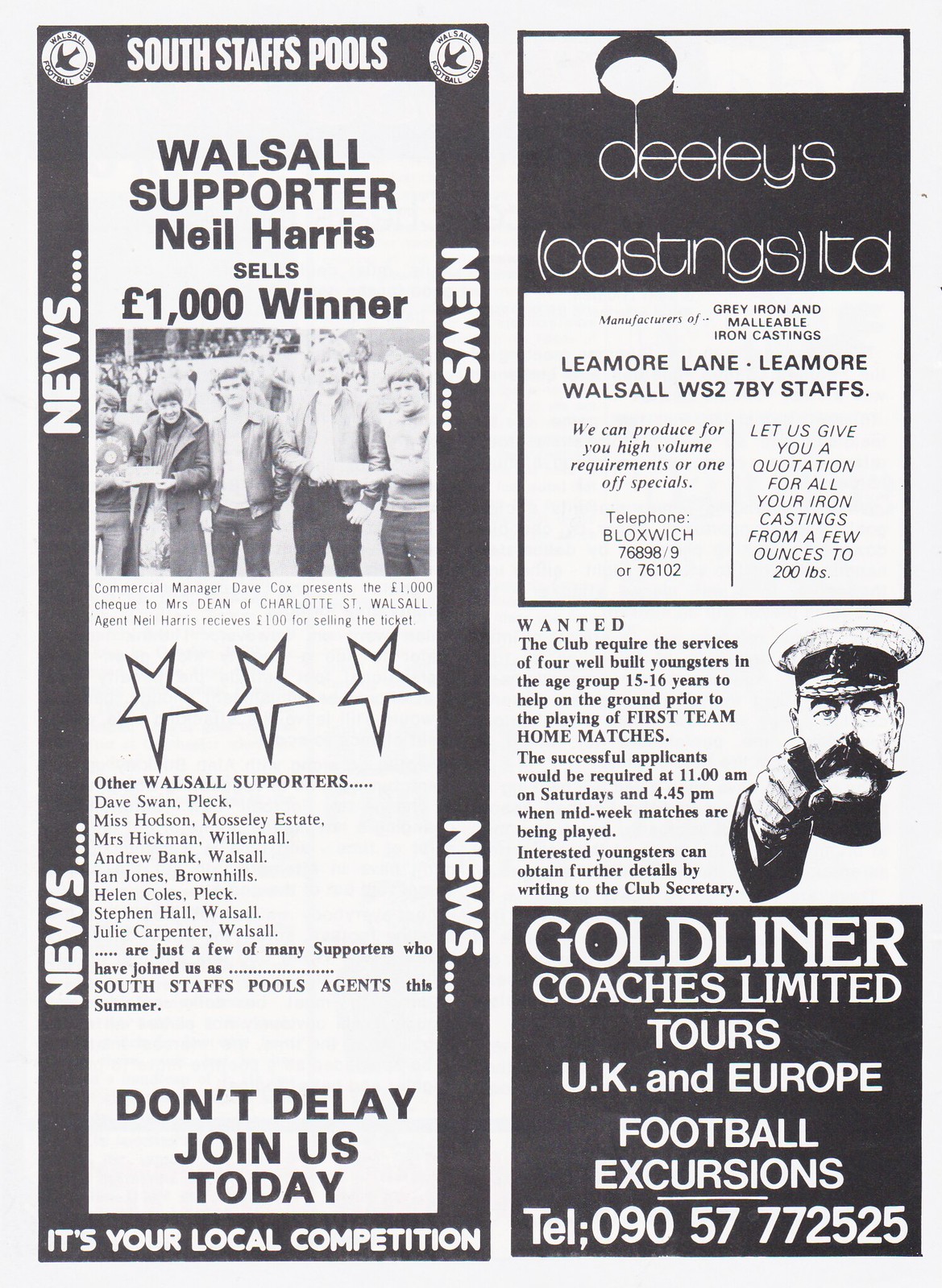The image is a black and white newspaper clipping bordered in black, featuring a variety of advertisements and notices. On the left side, it prominently showcases a heading "South Staffs Pools," below which is a headline stating "Walsall supporter Neil Harris sells $1,000 winner." Directly beneath this, there is a black and white photograph of five young men standing together. Further text underneath provides names and mentions they are Walsall supporters. At the bottom of this column, there is an exhortation, "Don't delay, join us today," and a note indicating it is a local competition.

The right column begins with the heading "Dealey's Castings LTD" and includes an advertisement box for Limor Lane, Limor, Walsall, WS2, 7 by Staffs. This ad offers quotations for iron castings of any weight from a few ounces to 200 pounds. Below this is a drawing of a man wearing a marine hat, pointing forward with a message to the left of the image seeking young workers, ages 15 to 16, to assist before first team home matches. At the very bottom, there is an advertisement with a black background and white letters that reads: "Gold Liner Coaches Limited Tours, UK and Europe, fall excursions." The advertisement also includes a telephone number: 0905-777-2525. The newspaper clipping is bordered by the word "news..." on the left and right sides.